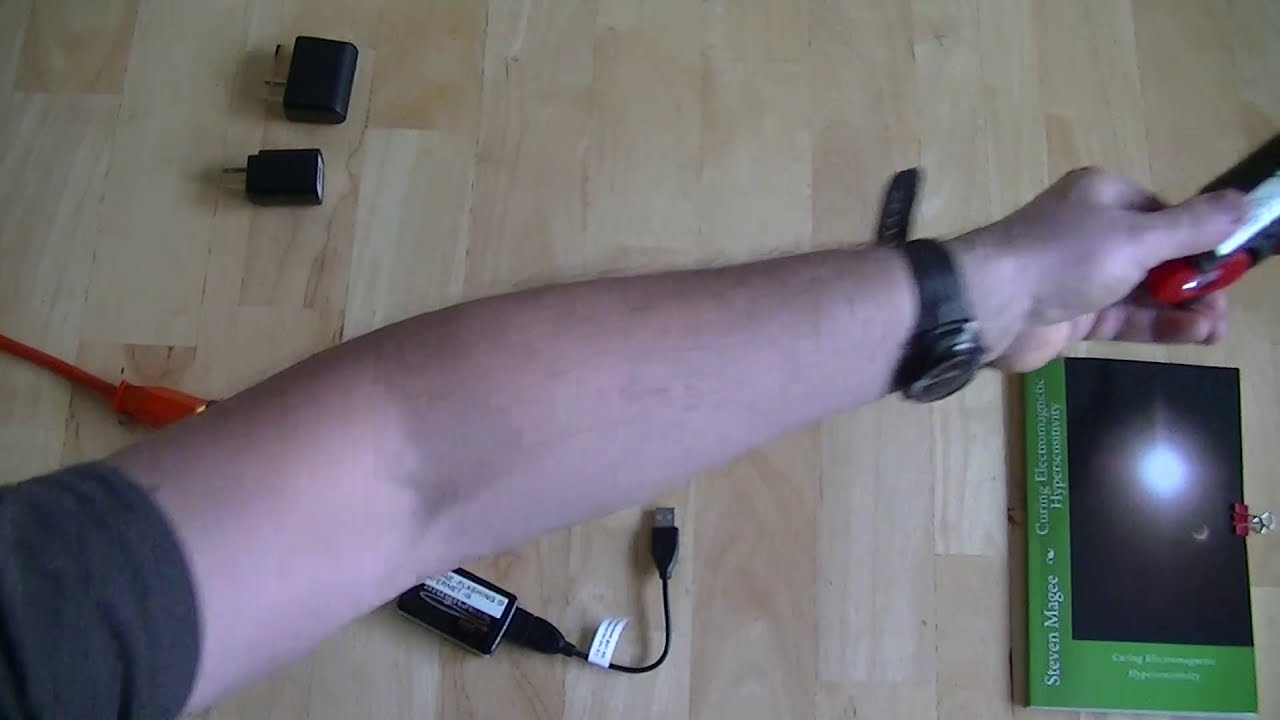A white person’s arm, partially covered in a black sleeve, stretches diagonally from the lower left to the upper right corner over a light wooden surface made up of small, untreated wood sections of varying shades. The arm wears an upside-down black wristwatch, with the dial visible against the palm. The hand grips a long, black cylindrical object with a shiny red point, the thumb positioned on top and the fingers grouped underneath. Around the arm, a variety of items are scattered. On the bottom right, there's a partially visible green and black book with the author’s name "Stephen McGee." The black section of the book features a radiant white sun in its center. A red clamp lies to the right of the book. Below the elbow, there's a USB adapter connected to a red extension cord. To the left of the hand, a red wire and a black USB cable extend. In the upper left corner, two black USB charging points rest on the wooden surface.